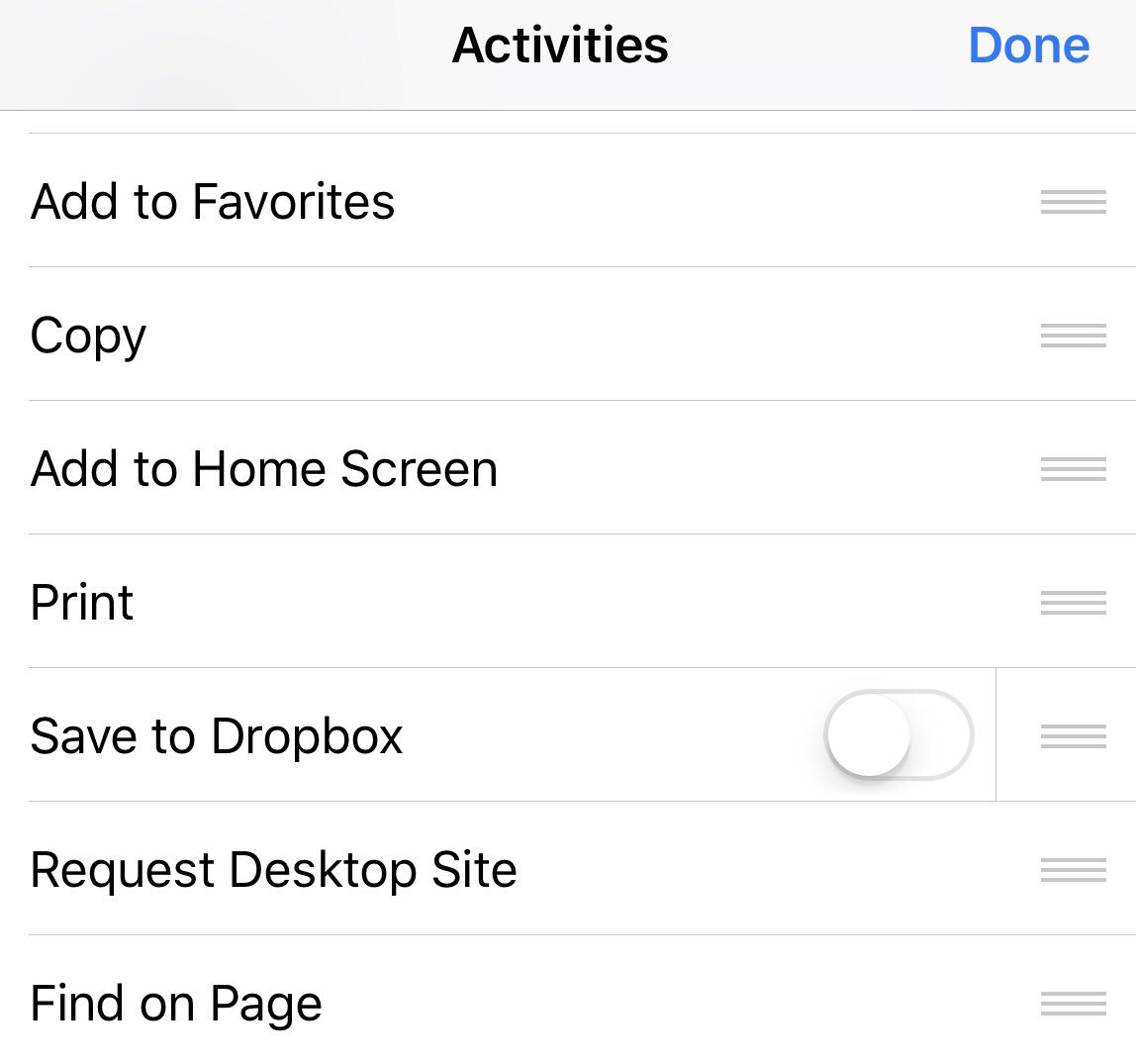The image displays a mobile device menu interface that consists of a vertically oriented rectangular layout. At the top, a light gray header bar features "Activities" in bold black text centrally aligned, with "Done" in bold blue text positioned on the right. Immediately below the header is a list of customizable options, each accompanied by a three-line "hamburger" drag handle on the far right, enabling users to reorder the items.

The listed options are: 
1. Add to Favorites
2. Copy
3. Add to Home Screen
4. Print
5. Save to Dropbox
6. Request Desktop Site
7. Find on Page

Each option is consistently styled with black text against a white background, except for "Save to Dropbox," which includes an additional on/off toggle switch located to the left of the hamburger drag handle. This interface allows for intuitive personalization, permitting users to arrange the activities based on their preference or priority.